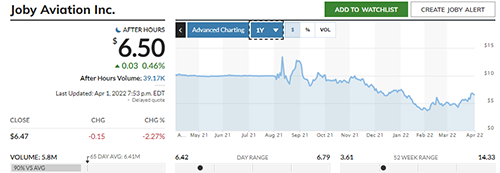This screen grab from a financial dashboard for Joby Aviation, Inc., showcases an after-hours trading snapshot with a colorful array of data points and graphs. The top of the screen features the company name "Joby Aviation, Inc." in black text. Just below it, there is a detailed breakdown of after-hours stock information.

One of the key graphics displays a blue crescent moon symbol adjacent to the after-hours trading price of $6.50, highlighted by an upward green arrow indicating a $0.03 increase, equivalent to a 0.46% rise. Below this, in blue text, the after-hours trading volume is listed as 39.17k shares. The timestamp for this data is noted as "last updated: April 1, 2022, 7:53 p.m. EDT."

The caption continues with information on the stock's performance at market close: the closing price was $6.47, with a change (C-H-G) of minus $0.15, reflecting a negative change percentage (CHG%) of -2.27%. It also references the 65-day average trading volume.

On the right side of the image, there's a graph with a white and gray background that charts the stock's performance from May 2021 to April 2022. The graph visually represents the fluctuations in the company's stock price with blue waves, providing a clear historical overview. Additional black text at the bottom likely includes further financial details and metrics.

This detailed screen grab offers a comprehensive view of Joby Aviation, Inc.'s stock performance during after-hours trading on April 1, 2022.